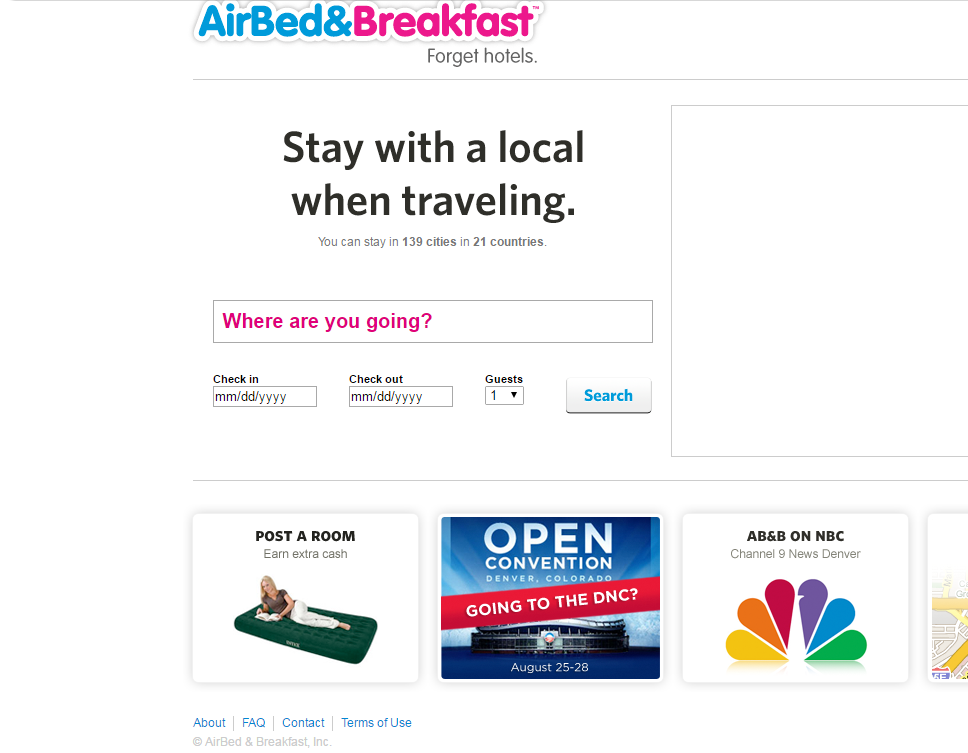The website prominently displays the phrase "Air Bed and Breakfast" in a blend of blue and pink, with the words "Air Bed and" in blue and "Breakfast" in pink. Below this title, a message in black letters encourages travelers to "Forget hotels. Stay with a local when traveling," and informs users that accommodations are available in 139 cities across 21 countries. Beneath this message, a search bar allows users to input their desired destination, prompted by the question "Where are you going?" in pink letters. 

Additional fields are provided for selecting check-in and check-out dates, where users can enter the day, month, and year. Adjacent to this, a "Guests" box allows travelers to specify the number of people accompanying them. The search functionality is completed with a "Search" button.

Further down the page, several advertisements are displayed. One ad encourages users to "Post a room, earn extra cash," and features an image of a lady lying on a mattress while reading a book. Another ad promotes the "Open Convention in Denver, Colorado," detailing the Democratic National Convention from August 25-28 with an image resembling a cruise ship. Additionally, a note mentions "ABNB on NBC Channel 9 News Denver."

At the bottom of the page, links to "About," "FAQ," "Contact," and "Terms of Use" are provided, along with a note indicating that the content is copyrighted by Air Bed and Breakfast Incorporated.